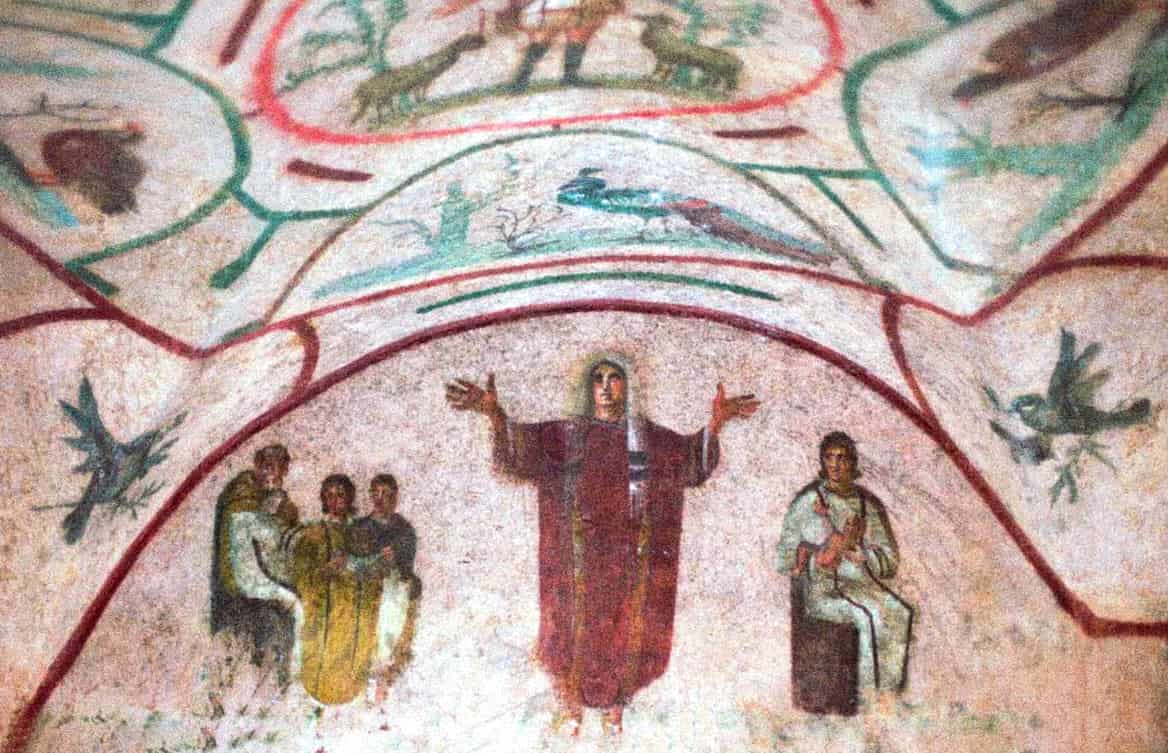The image depicts a vibrant and intricate painting on a church ceiling, potentially a fresco or mosaic with a multicolored and detailed composition. At the center bottom, a figure believed to be Christ is depicted in a red robe with outstretched arms, wearing a white scarf with black stripes and fringe. To Christ's right, a man in a white robe with black trim is seated on a dark, brown chair with his hands in prayer. On Christ's left, there are three individuals: a priest in a white robe with a yellow cape, a woman in a yellow dress, and another person of indeterminate gender wearing a blue shirt and white pants.

The painting is surrounded by various panels showcasing colorful birds and other elements. On the right side of the image, a bird is portrayed mid-flight within a circled area, set against a backdrop of red and green lines, depicting another bird and a tree. At the very top, there is the bottom half of a person with knee-high boots and a couple of sheep, situated in a large red circle with trees on either side. Additionally, a peacock with a long tail, another bird, and a bush are depicted within smaller arched areas. The overall artwork is intricate and beautifully detailed, capturing a rich tapestry of religious and natural symbolism.